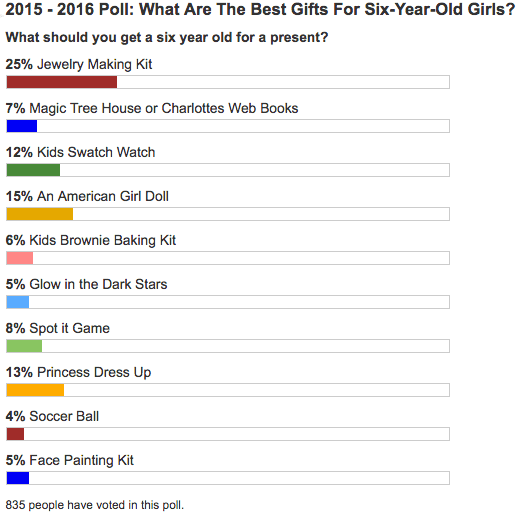Here is a cleaned-up and detailed caption for the image:

---

The image depicts a screenshot of an online poll conducted in 2015-2016, titled "What are the best gifts for 6-year-old girls?" The poll asks participants what they believe would make the ideal present for a 6-year-old girl. The most popular choice, attracting 25% of the votes, is a jewelry making kit. Below this, the options are listed with individual colored bars representing their respective percentages of total votes: 

- Magic Tree House and Charlotte's Web books: 7%
- Kids Smart Watch: 12%
- American Girl Doll: 15%
- Kids Brownie Baking Kit: 6%
- Glow in the Dark Sticker Stars: 5%
- Spot It Game: 8%
- Princess Dress Up: 13%
- Soccer Ball: 4%
- Face Painting Kit: 5%

At the very bottom of the poll, small text indicates that a total of 835 people participated in the voting.